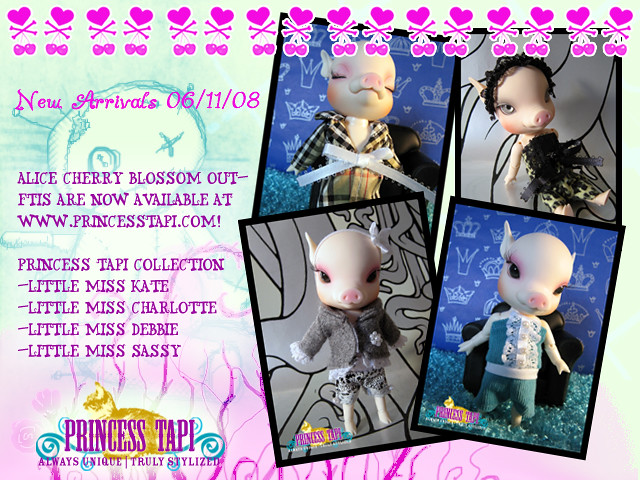This vibrant advertisement features an alluring blend of colors, transitioning from a light greenish-blue at the top to a soft pink at the bottom. Dominating the top section, a decorative row of hot pink hearts, crossbones, and dangling cherries create an eye-catching border. To the left, prominent pink text announces "New Arrivals 06-11-08" with "Alice Cherry Blossom outfits now available at www.princesstoppy.com." Beneath this, it highlights the Princess Toppy Collection, featuring Little Miss Kate, Little Miss Charlotte, Little Miss Debbie, and Little Miss Sassy. The right side showcases four richly detailed images of pig dolls dressed in fashionable outfits, such as a gray jacket edged in white lace and a teal tank top adorned with white lace. Intricate teal swirls and wiry pink lines embellish the golden cat icon positioned at the bottom left. Finally, in capital letters, the whimsical tagline reassures, "Princess Toppy, Always Unique, Truly Stylized."